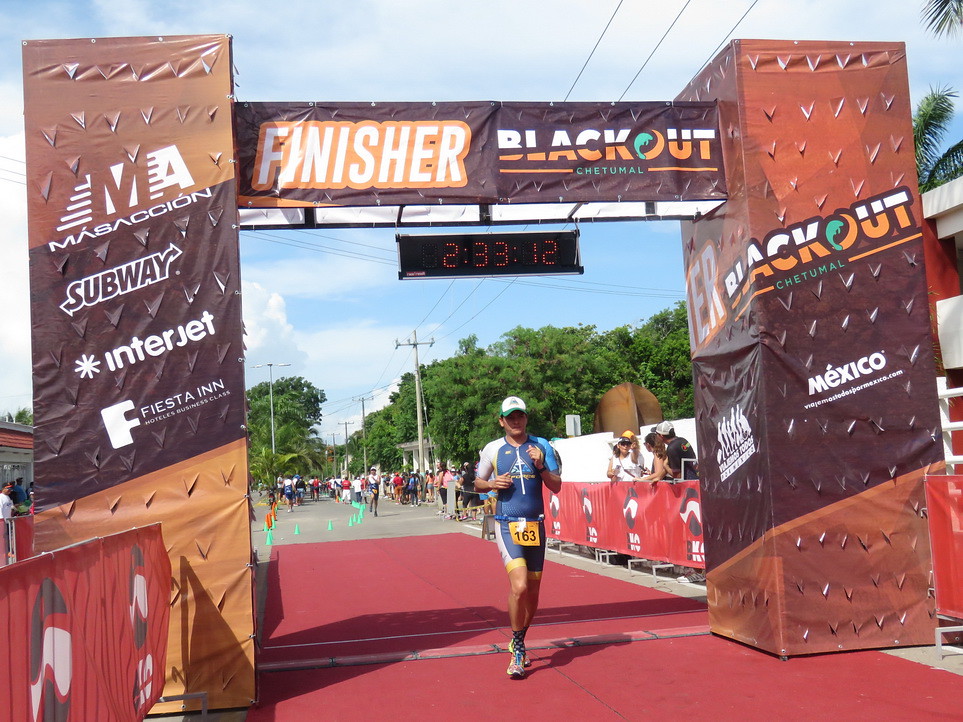The image captures the climactic moment of a running race's finish line, prominently displaying a distinctive finish structure composed of two rectangular brown pillars connected by a horizontal bar. A vibrant red mat marks the finish line. Above the structure, a digital timer indicates a completion time of 2 hours, 33 minutes, and 12 seconds. The horizontal bar features a "Finisher" banner with the word "blackout" alongside "Chetumal," suggesting the location or event name.

In the foreground, a runner sporting bib number 163 is making his final strides across the finish line. He wears a white cap and a blue jersey, paired with sneakers. Sponsors' logos - including Subway, Interjet, Fiesta Inn, and EMA Massassi - adorn the pillar on the left, while "blackout" and "Chetumal Mexico" are displayed on the right. The background teems with spectators and other runners heading towards the finish line. The setting is bright and lively, with blue skies, scattered clouds, telephone wires, and abundant green trees, accentuating the scene with a burst of colors, including black, white, gray, green, orange, red, yellow, blue, mint green, and gold.